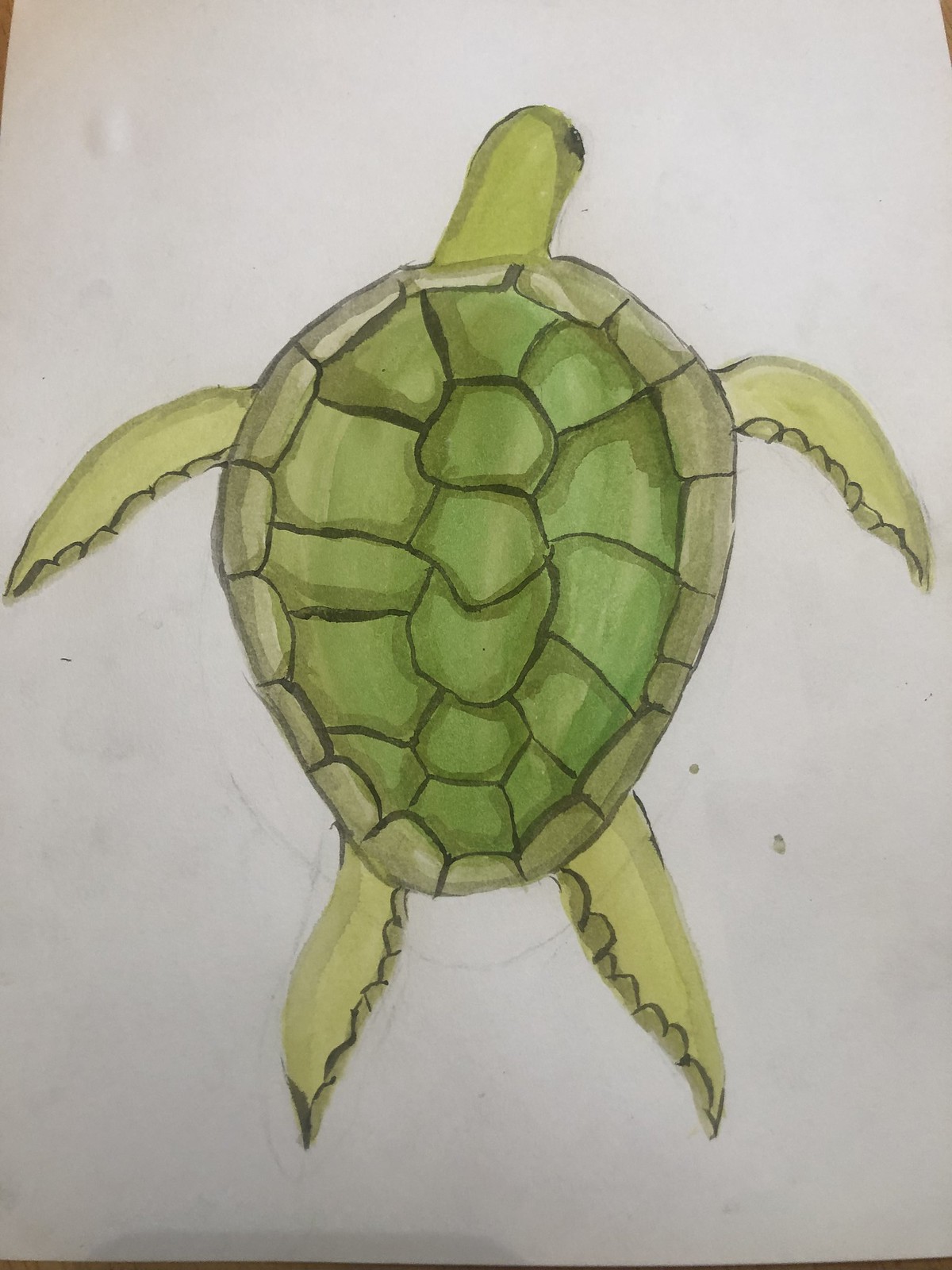This photograph captures a hand-drawn image of a sea turtle, set against a background that suggests it was taken over a table with a brown hue. The turtle drawing is on standard white paper, visible edges at all four corners indicating the paper's boundary. The turtle, possibly rendered by an older child, embodies a detailed yet simplistic style. Its head is oriented away from the viewer, and it has four flippers, consistent with sea turtle anatomy. The shell is colored in varying shades of green, with the darkest hues accentuating the ridges and segments. The flippers are depicted in a lighter green, while the shell's outer edges are highlighted with brown segments. Despite the absence of a water backdrop, the drawing conveys the subject's aquatic nature effectively.